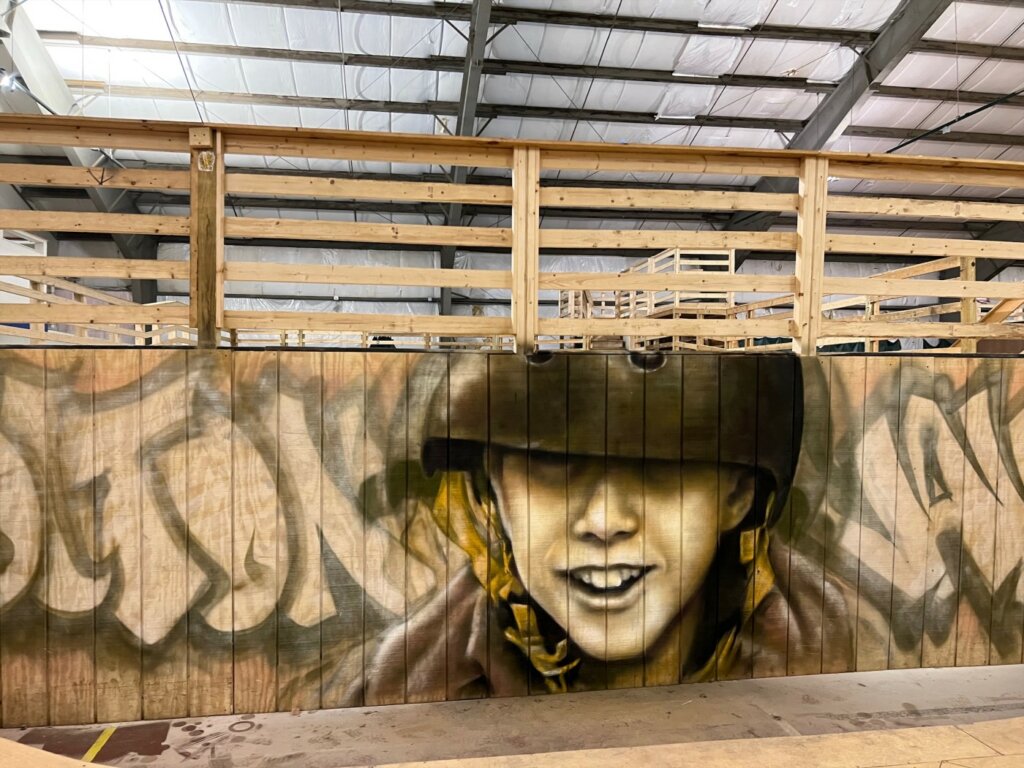The image depicts the interior of what appears to be an indoor skate park. Dominating the scene is a large brown wooden fence, which serves as a backdrop for a striking mural. This mural features the face of a young boy wearing an oversized black helmet, secured with a yellow chin strap. The boy's eyes are obscured by the helmet's size. Surrounding the central image are various graffiti tags, with discernible letters such as T-O-N on one side and N-A or possibly W on the other.

Above, the structure reveals a gray metal frame supporting a partially translucent roof, likely made of dark gray or black plastic or glass panels. The flooring is a concrete surface, partly covered with black graffiti paint drips. Additionally, the wooden elements of the fence are constructed from horizontal boards and placed atop a lighter brown wooden base, similar to 2x4s. This space is likely designed for skateboarding, evidenced by the wooden ramps and structures that compose the skate park, offering a rugged, urban aesthetic to the indoor environment.